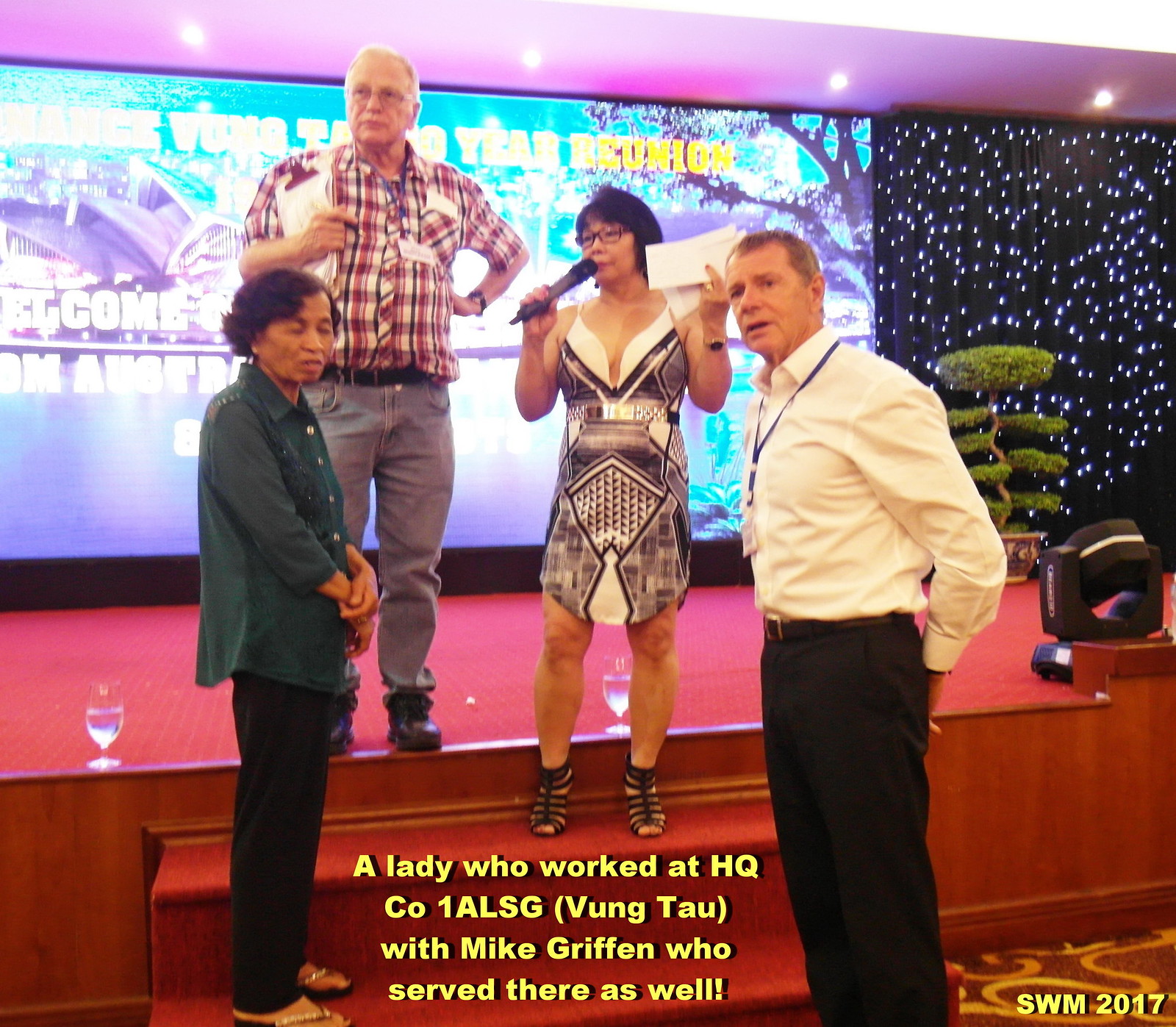The image captures a group of four people on a red stage with a large TV screen in the background displaying the word "REUNION" amid a starry, black-and-white pattern. The group consists of two women and two men, all wearing lanyards with their names and perhaps other details. The two women are dressed more formally. One woman appears to be in a character suit, holding a piece of white paper and a microphone. Next to her stands a casually dressed man in a plaid shirt, holding a board with papers. Another man, in a plain button-up shirt, pants, and sandals, stands on a step below them, looking down. To his right stands the fourth person, dressed in a white shirt and dress pants with a badge around his neck, possibly indicating his managerial role. Yellow lettering at the bottom of the image mentions the HQ company and specifically names a lady who worked there alongside Mike Griffin, suggesting this may be a reunion of former colleagues. Lighting equipment is visible above them, adding to the formal backdrop of the event.